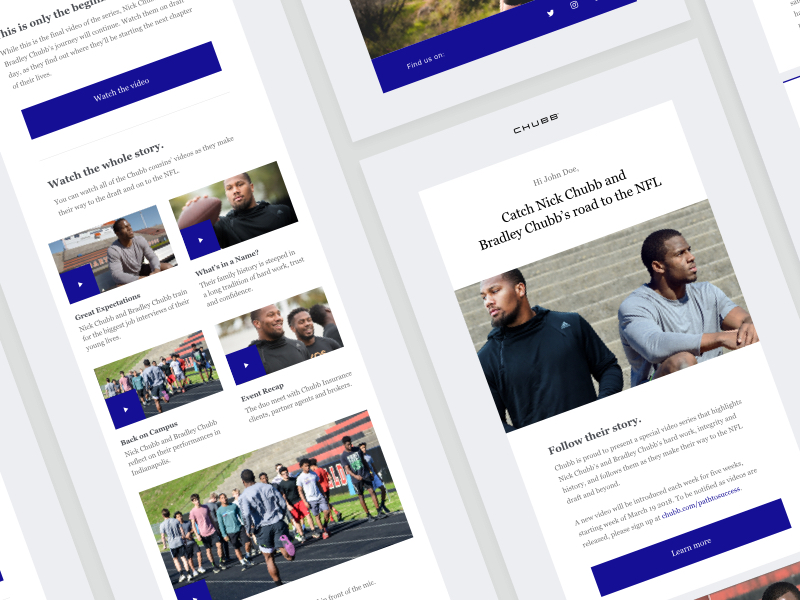**Brochure Caption: The Journey of Nick Chubb and Bradley Chubb**

This detailed brochure captures the captivating journey of Nick Chubb and Bradley Chubb as they prepare for their entry into the NFL. The title "This is Only the Beginning" sets the tone, emphasizing that while this is the conclusion of a video series, it marks the start of an exciting new chapter in their lives. Below the title is a blue rectangular button inviting viewers to "Watch the Video."

Continuing, a prominent heading invites viewers to "Watch the Whole Story." Underneath, the brochure lists four compelling videos that showcase their path to the draft:

1. **Great Expectations** - Nick Chubb and Bradley Chubb train for the biggest job interviews of their young lives.
2. **What's in a Name?** - A deep dive into their family history, revealing a legacy of hard work, trust, and confidence.
3. **Back on Campus** - Reflections on their performances and experiences in Indianapolis.
4. **Event Recap** - The duo’s interactions with Chubb insurance clients, partners, agents, and brokers.

Accompanying these descriptions is an image of a track and field, paired with a greeting that reads, "Hi, John Doe." The heading next to the image, "Chubb," promotes their journey with the subtitle, "Catch Nick Chubb and Bradley Chubb's Road to the NFL." A picture of the athletes is included, followed by the heading "Follow Their Story." This section reveals that Chubb is proud to present a special video series highlighting their hard work, integrity, and history as they march toward the NFL draft. A new video is released weekly for five weeks, beginning March 19, 2018. Readers are encouraged to sign up for notifications at chubb.com/pathtosuccess.

To sum up, the brochure concludes with a rectangular blue box inviting readers to "Learn More." 

This comprehensive caption gives a vivid and thorough depiction of the brochure's content, seamlessly guiding the reader through the journey of Nick and Bradley Chubb.